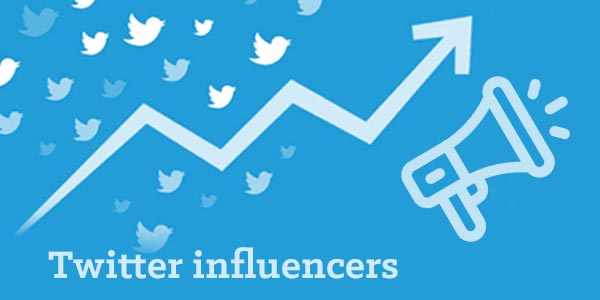In the image, a blue rectangular banner forms the background. Within this blue space, there are several white Twitter bird icons, symbolizing the social media platform. A jagged line graph overlays the background, likely indicating data trends or metrics related to Twitter activity. Below the graph, the text reads "Twitter Influencers" in a bold and clear font. On the right side of the image, a detailed illustration of a megaphone is shown, complete with a grip and trigger. Sound lines are emitting from the megaphone, suggesting the amplification of messages, representative of influencer reach or broadcast power. The overall color scheme prominently features various shades of blue, reinforcing the Twitter theme. This detailed infographic is designed to convey information about the impact and reach of Twitter influencers.